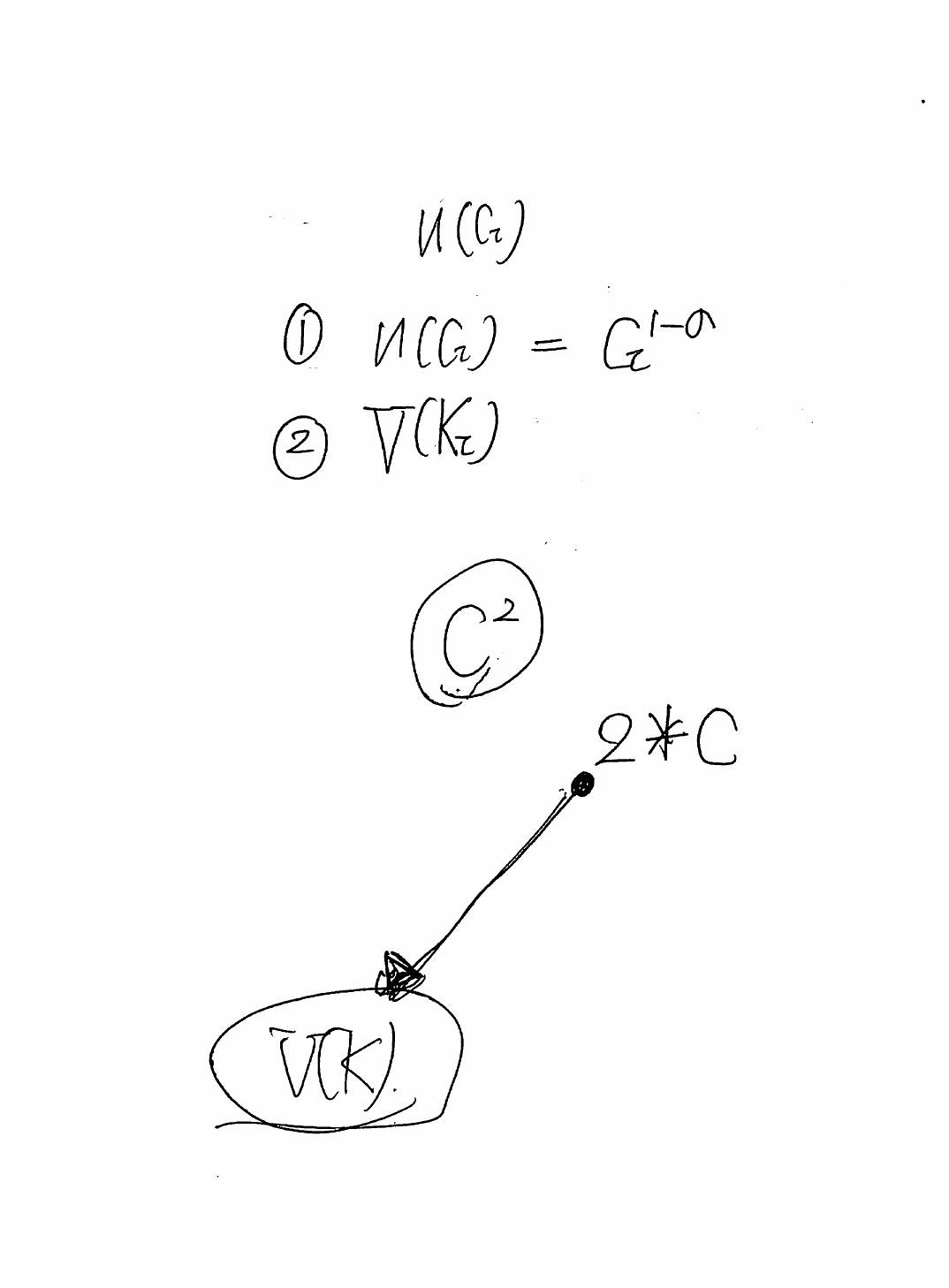This image appears to be a scanned copy of handwritten notes, characterized by black, somewhat pixelated text that resembles a natural handwriting style. The topmost section features the notation \( U(C_2) \), with a subscript ‘2’ between parentheses. In the row below this, there is a circled ‘1’ followed by \( U(C_2) = C_2^{1-0} \), where '1-0' is written in superscript. 

Continuing to the next row, a circled ‘2’ is initially present, succeeded by an upside-down triangle or ‘V’ symbol incorporated within parentheses as \( V(K_2) \). Below these entries lies a \( C^2 \) circumscribed by a circle. Diagonally downward to the right of this is a sequence consisting of ‘2’, an asterisk or star symbol, and ‘C’. Notably, there is a black dot proximal to the ‘2’, from which thick black lines extend, culminating in the heavily shaded triangular point of an arrow.

In a large, encompassing circle situated nearby, the lettering \( V(K) \) is discernible. The overall layout and specific mathematical notations suggest this is a diagrammatic or formulaic representation, possibly from a scientific or mathematical context.